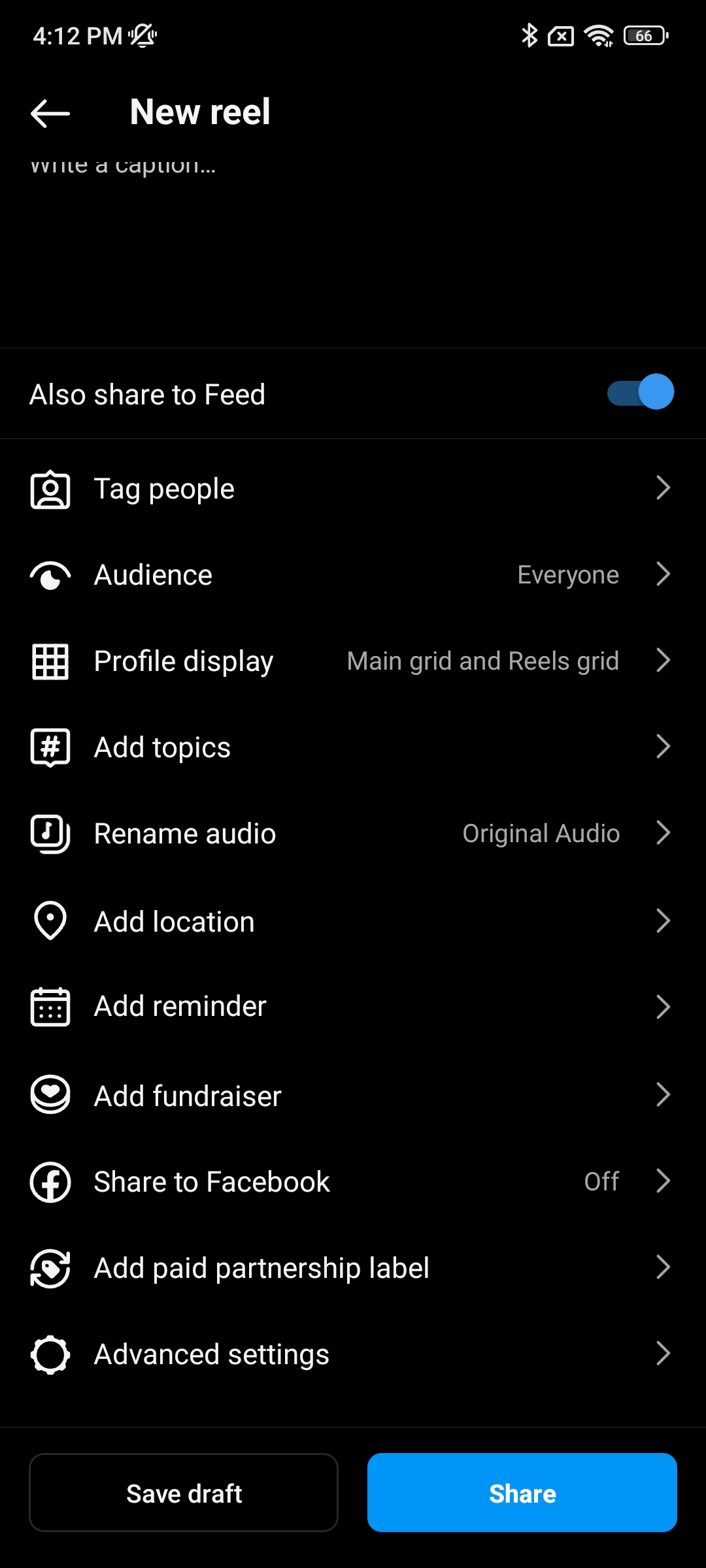A screenshot of an Instagram interface on a black background, captured at 12:14 PM. The screen displays the "New Reel" menu with several interactive elements and settings. An arrow points to the left, indicating a navigation option. The interface is shared to the feed, with a toggle bar turned on. Several sections, including "Tag People," "Audience," "Profile Display," "Main Grid," "Reels Grid," "Add Topics," "Rename Audio," "Provisional Audio," "Add Location," "Add Reminder," "Add Fundraiser," "Share to Facebook," "Add Paid Partnership Label," and "Advanced Settings," each feature a greater-than symbol (>) to the right, suggesting additional options or subsections.

"Audience" is set to "Everyone." 

At the bottom of the screen, two buttons are displayed: a black rectangle labeled "Save Draft" in white text, and a blue rectangle labeled "Share" in white text.